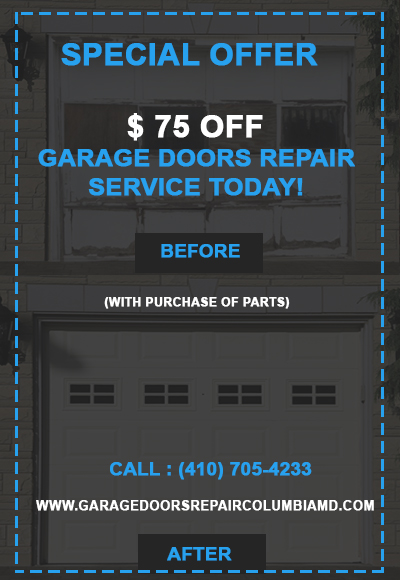The image in question is a screenshot of an advertisement featuring a vertically oriented design. The background consists of two identical photos depicting the front of a standard garage door, arranged one on top of the other to create an elongated look. However, these images are somewhat obscured by a translucent gray overlay, making it difficult to discern specific details or colors of the garage doors themselves.

Overlaying the background is a text-laden gray square, which is central to the advertisement's message. The ad employs a design element often seen in coupons, with a dotted-line border giving it a distinct "coupon-like" appearance. The main text in blue reads: "Special Offer: 75% Off Garage Doors Repair Service Today." Additional information clarifies that this offer is valid with the purchase of parts. The ad also includes a phone number, a website, and features two boxed sections labeled "before" and "after," which appear to function as buttons.

Overall, the ad's visual elements and text are designed to catch the viewer's attention with a significant discount, while ensuring essential contact details and conditions of the offer are easily accessible.